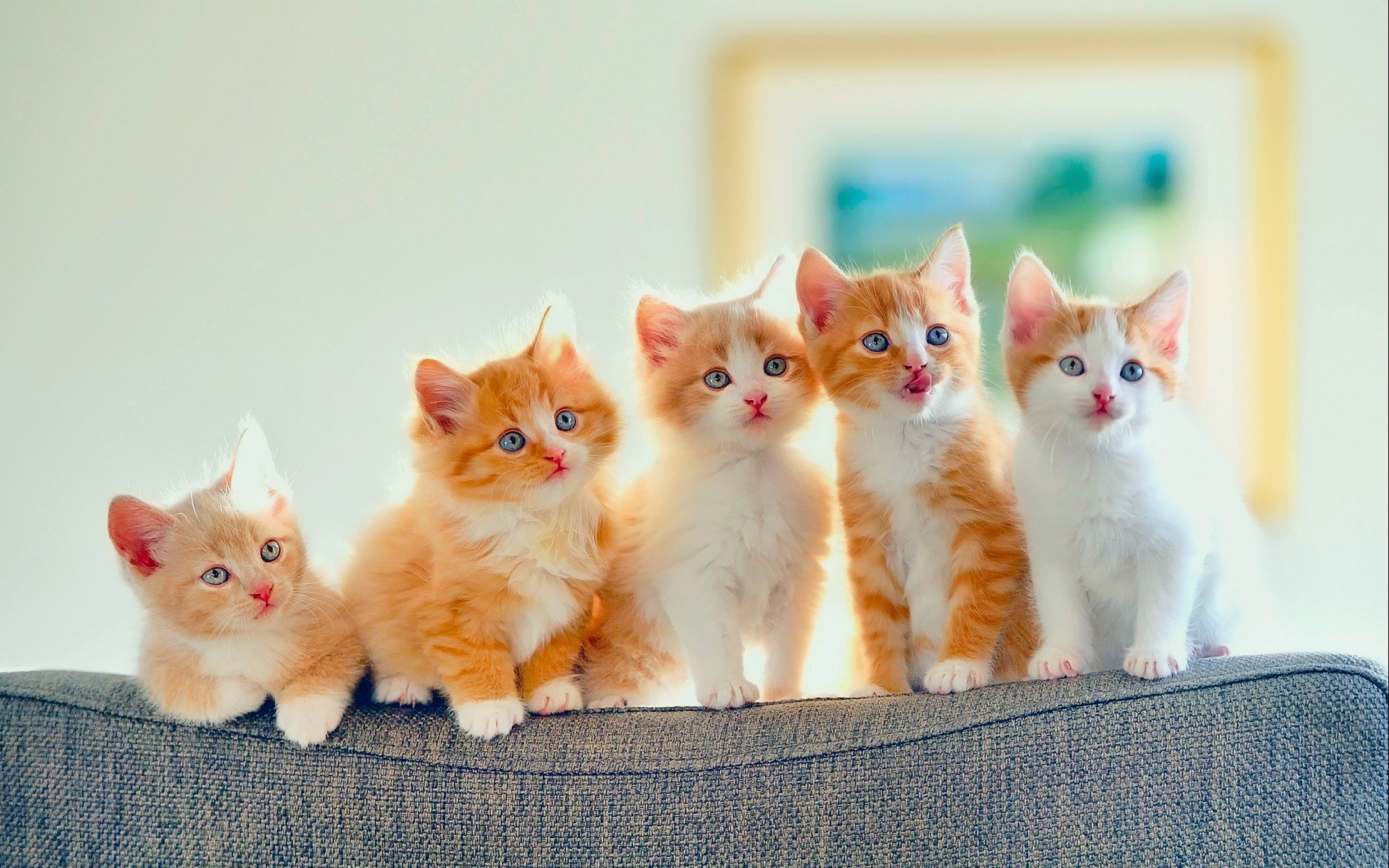In this detailed image, five tiny kittens are perched atop the back of a blue, textured couch, each gazing towards the right. The leftmost kitten appears to be dangling with only its front paws visible, one arm bent and the other holding on, its light orange fur and pink nose accentuated by sunlight. Adjacent to it is an orange and white kitten with blue eyes and a particularly fluffy coat. The next kitten, similarly colored, has a predominantly white chest and legs complemented by slightly less vibrant blue eyes. Following is another orange and white kitten, featuring distinctive tiger stripes and a playful pose with its tongue sticking out. The final kitten is mostly white with patches of orange around its ears, characterized by striking blue eyes and a pink nose. All five kittens have pointed ears, pink noses and mouths, and light blue eyes with small black pupils. The background reveals a blurred painting framed in gold with a white mat, showcasing hints of blue and green hues, set against a barren white wall.